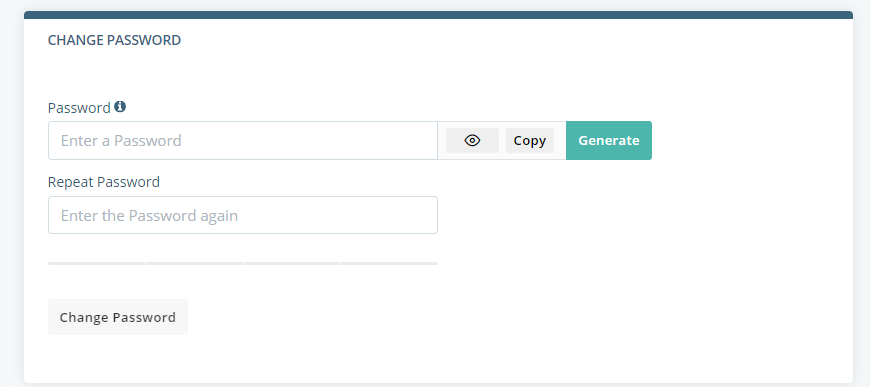The image depicts a straightforward "Change Password" interface within a clean, white rectangular box. At the very top, the box is labeled with "Change Password" in bold text. Below this header, two password input fields are prominently displayed. The first field is labeled "Enter a Password," and the second, directly underneath it, is labeled "Repeat Password." Both password fields feature icons on the right side: an "eye" icon to toggle password visibility, and a "copy" button to duplicate the text.

Adjacent to these fields is a vibrant turquoise button with white text that reads "Generate," offering users an option to create a secure password automatically. At the bottom of the box is a functional "Change Password" button, prompt for submission.

Aesthetically, the interface is minimalistic and user-friendly, utilizing a palette of white, blue, gray, and black. The top of the white box is accentuated by a navy blue design bar that spans its width, adding a touch of color contrast and visual structure. The input fields are currently empty, indicated by placeholder text instructing users to "Enter a Password" and "Repeat Password." There are no additional decorative elements or complex features, enhancing the simplicity and clarity of the layout. Overall, the design serves its purpose effectively, making it easy for users to change their password without any confusion or distraction.